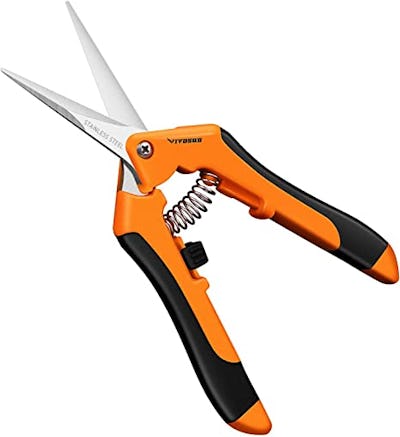This detailed image depicts a robust cutting tool, specifically a pair of spring-loaded scissors. The scissors feature two sharp triangular blades made from stainless steel, each inscribed with "stainless steel" and joined together by a central screw. The ergonomic handles are predominantly orange, accented with black on the outer edges for enhanced grip and comfort. A prominent silver spring is positioned between the handles, facilitating the cutting motion by keeping the blades open when not pressed together. On the left handle, there's a small black tab designed as a safety lock to clasp the blades closed when not in use. Additionally, a slider mechanism on the bottom handle adjusts the blade's operational angle, acting as a stopper to control the depth of the cut. The background of the image is plain white, drawing full focus to the tool's detailed features and design, currently displayed in an open position. The inscription "VIVO500" can be discerned on one of the handles, likely indicating the model or brand.